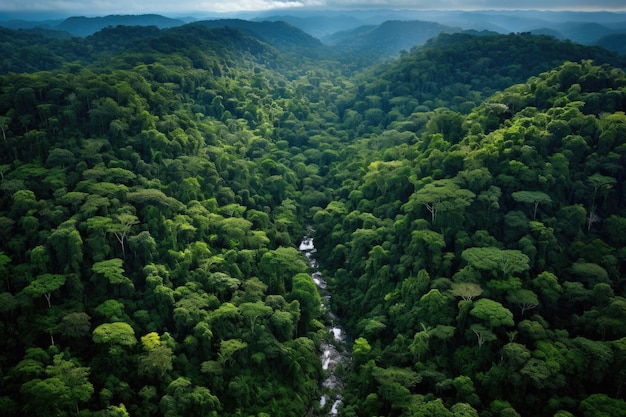This breathtaking aerial photograph appears to be taken from a high vantage point, possibly from a helicopter or the peak of a mountain, showcasing a vast and verdant forest that extends endlessly into the distance. The landscape is dominated by a seemingly infinite expanse of lush green trees with skinny trunks, their vibrant canopies creating a mesmerizing, wave-like pattern across undulating hills that resemble mountains from afar. In the heart of this dense forest, a winding river or brook cuts through the greenery, adding a fluid, dynamic element to the tranquil scene. The sky above is a gentle blue, dotted with white, fluffy clouds and slightly veiled by a mist or fog, which softens the horizon and enhances the rich, almost surreal quality of the colors. The interplay of sunlight and shadow across the treetops and the overall serene atmosphere of the image suggests it was taken during daylight hours, contributing to the dreamlike and pristine beauty of this forested landscape.